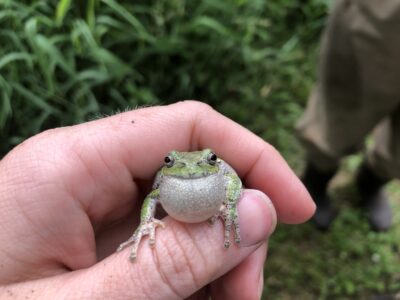In the photograph, a Caucasian left hand emerges from the bottom left corner, delicately holding a small green frog. The frog, which appears ready to croak, has its throat inflated like a bubble, giving the impression of an impending "ribbit." The amphibian's tiny limbs rest on the person's thumb, appearing diminutive next to the thumb's size. The detailed foreground contrasts with a blurred background of tall, green grass and weeds. Off to the right, partially obscured but clearly visible, are a pair of legs clad in khaki pants and black boots, suggesting a scene set outdoors, perhaps in a jungle or a grassy field. The overall setting appears to be in the morning, adding a subtle, fresh ambiance to the image. The frog, with its silvery underside and prominent green hue, stands out as the focal point, while its gaze is directed either at the photographer or the person holding it. The absence of text allows the vibrant colors and natural elements to speak for themselves.